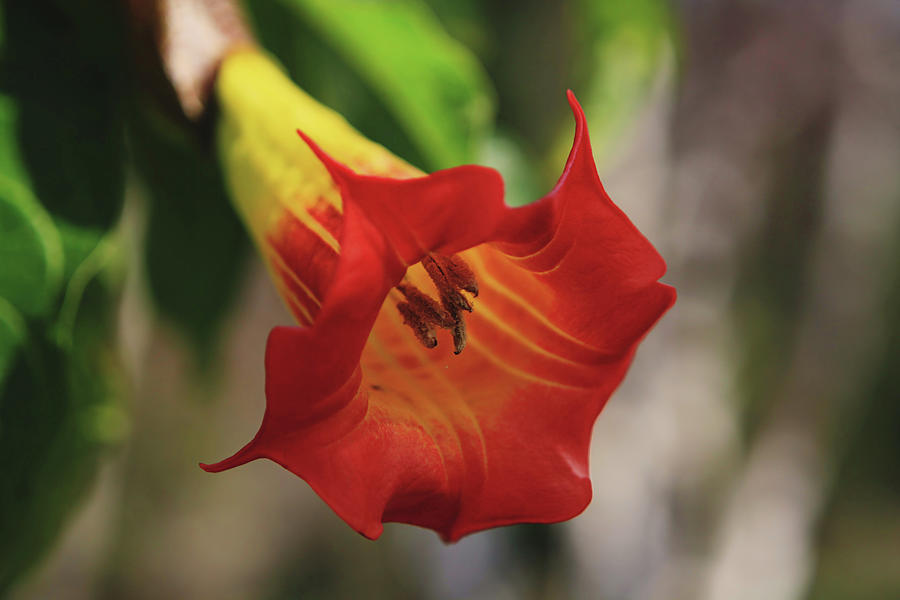This photograph showcases an up-close and detailed image of a striking flower. The flower displays rich red-orange petals that curl back, creating a bell or cone-shaped bloom. The petals fade towards a yellow hue at the base, where you can observe four red, fuzzy pistils emerging from the center. The inner area of the flower reveals yellow pod-like structures that house seeds and pollen.

The photograph captures the flower in hyper-focus, emphasizing its vivid colors and delicate textures. The background, featuring green leaves and stems, is blurred out, rendering it indistinguishable and maintaining the viewer’s attention on the flower's intricate details. The overall coloration transitions smoothly from a predominant red-orange to a yellow, illuminated subtly by natural sunlight, which casts a gentle highlight on the lower part of the bloom. This composition, with its profound clarity and vibrant palette, celebrates the exquisite beauty of the flowering plant.